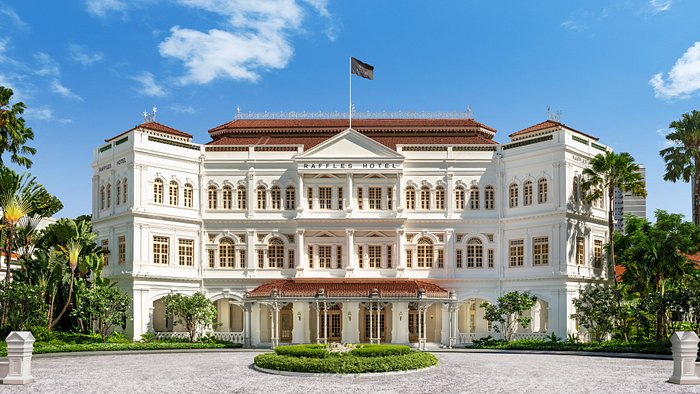The photograph captures the majestic Raffles Hotel, a grand three-story white colonial building, adorned with red terracotta tiles that give it a tropical flair. The hotel's name, "Raffles Hotel," is prominently displayed at the top, beneath a flagpole that stretches towards a sunny sky dotted with a few wispy clouds. Surrounding the hotel, lush green landscaping includes a circular driveway of gray concrete, featuring a central garden area with well-manicured bushes. Framing the scene are vibrant green trees and towering palm trees, creating an inviting and serene atmosphere. In the backdrop, modern buildings peek through, adding a contrast to the colonial charm of the hotel. Notably, decorative white statues or objects can be seen at the far left and right sides, enhancing the hotel's elegant allure.